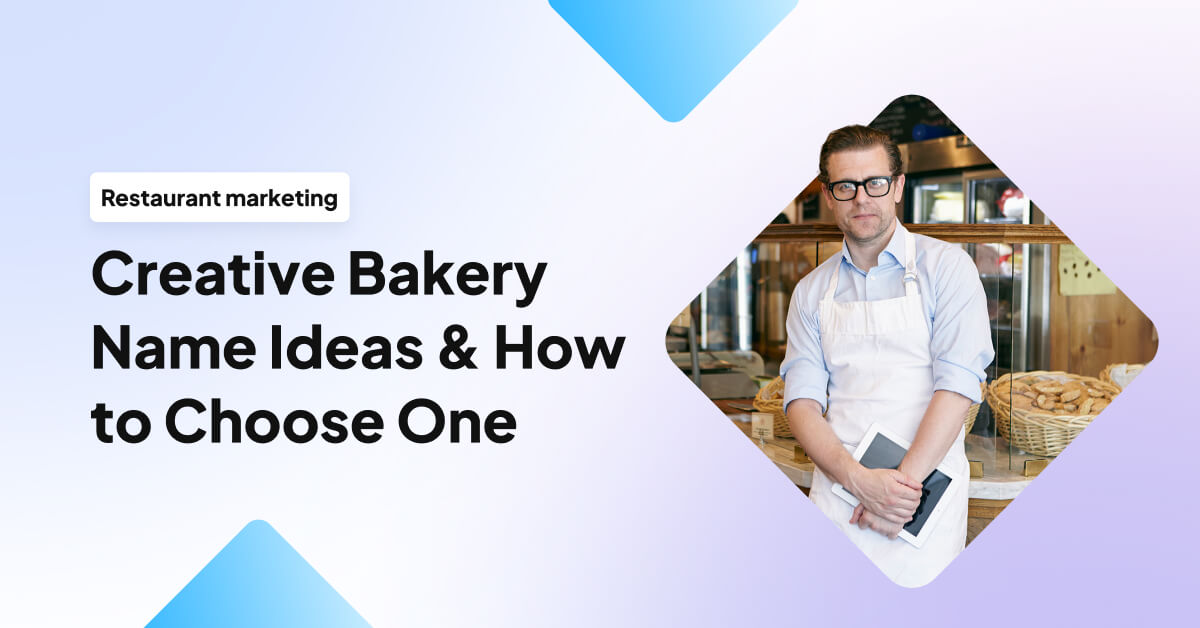The image is a detailed advertisement for a bakery-themed restaurant marketing class. The background transitions from light purple to pinkish tones, with three prominently placed blue triangles: one at the top, one in the middle, and one at the bottom left, pointing upwards. On the left side of the image, a text box with black lettering reads: "Restaurant Marketing," followed by larger text stating: "Creative Bakery," and continuing with: "Name Ideas and How to Choose One."

On the right side, within a diamond-shaped cutout, stands a man dressed as a chef. He is wearing a light blue button-down shirt with the sleeves rolled up, a white apron, and black-rimmed glasses. He holds a tablet close to his body. Behind him is a setting of a bakery, with visible kitchen items, baskets of food, and baked goods. A cabinet and a cash register can also be seen in the background, adding to the authentic bakery atmosphere.